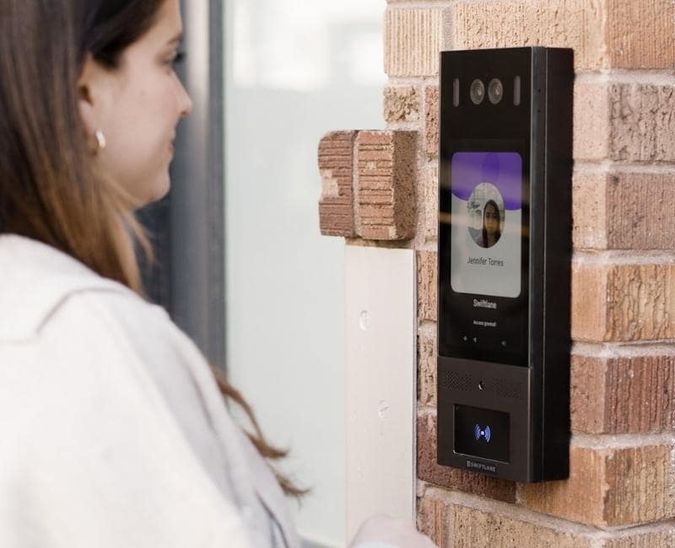The image depicts a high-tech smart camera system mounted on a dull red-brown brick wall near a window with a white curtain and a dark gray frame. The device has two camera lenses at the top and a screen below, which displays an image of a woman in a white hoodie with gold earrings, identified as Jennifer Torres. The screen is divided into blue and white sections, with a circular area displaying Jennifer's image and her name in black text. At the bottom of the device, there are blue indicator lights and icons suggesting Wi-Fi connectivity and battery status. The woman stands to the left side of the frame, looking at the screen, engaging in what appears to be a conversation through this sophisticated video doorbell system.